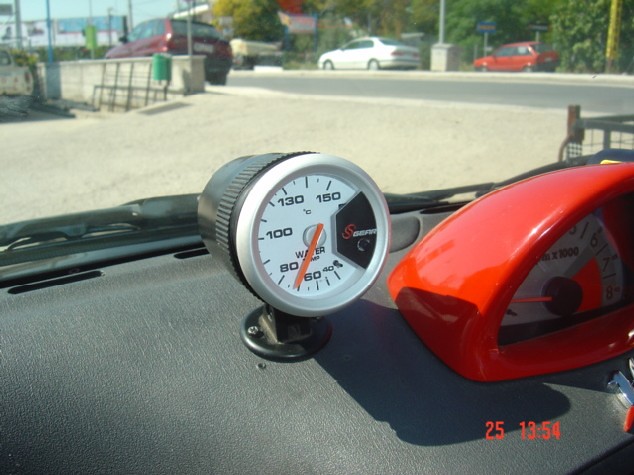The image captures a time-stamped photograph, recorded at 25:13:54, taken from inside a car. The main focus is on two distinct gauges on the car's dashboard. The first gauge, circular in shape, ranges from 40 to 150 and is currently indicating 70, marked by a red line. The second gauge, more triangular in form, appears to scale from 1 to 8, though readability is partially obscured, it registers at 1.

Visible through the car window, a fence is positioned to the right. Beyond the fence, a street is visible, lined with several trees and interspersed with a few cars. A green highway sign with white writing is noticeable further ahead, alongside multiple streetlight poles and a trash can, adding to the urban setting of the scene.